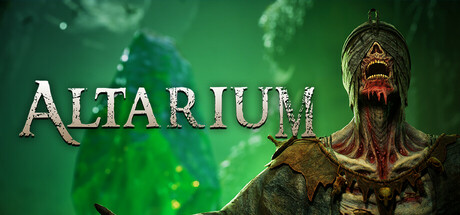This image showcases a detailed crest-like emblem set against a metallic black background with numerous light gray scratches. Dominating the center is a circular badge with a slightly weathered, matte metallic texture, accentuated by a thin silvery outline. Sticking out from the circle are various misshapen points: three at the top, two on each side, and two at the bottom. Encircling the emblem's center, the phrase "Trudit Non Ducit Fatum" is inscribed in three-dimensional lettering, mirrored and repeated upside down at the bottom.

Within the circle, a vivid red, wax seal-like design forms the backdrop for a jagged silvery triangle resembling an "A" with spikes protruding from it. Superimposed on the triangle in white text is the word "Alterium." The intricate details and the classical Latin phrases suggest a noble or ancient theme, possibly linked to a fictional universe or video game due to the stylistic elements and the bold, futuristic font used for "Alterium." The emblem’s weathered stone-colored look and cracked texture, juxtaposed against the dark, scratched background, enhance its aged and storied appearance.